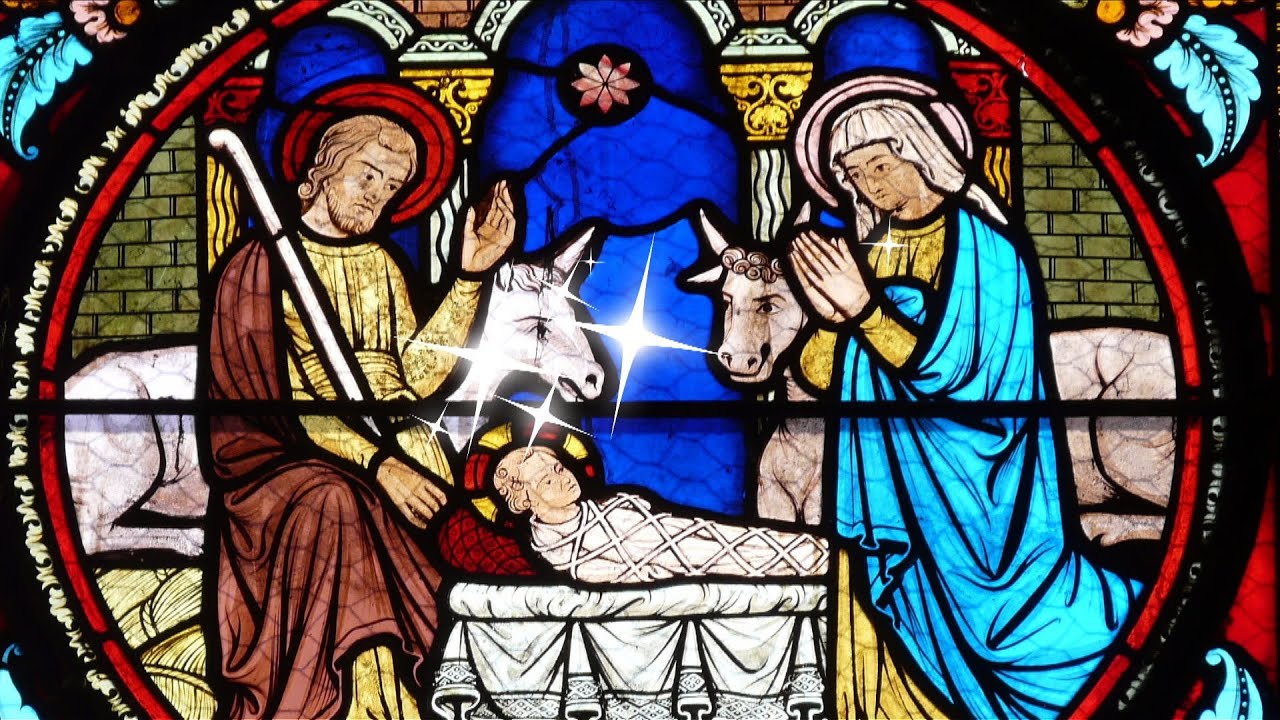This vibrant stained glass depiction of the nativity scene captures a deeply detailed and colorful representation of the birth of Jesus. At the center of the oval image, baby Jesus lies in a creche, swaddled in white with a red and gold halo. To the left, Joseph gazes down at him, his left hand raised above the child, while his right hand holds a staff. Joseph, dressed in a brown cloak and yellow robes with a red halo, obscures part of a donkey, whose head and back are faintly visible. To the right, the Virgin Mary, adorned in blue robes with a white veil and halo, kneels in prayer, her eyes fixed lovingly on her son. Behind Mary, the head and back of a cow can be seen, adding to the serene rural backdrop. Surrounding the central scene, the stained glass features intricate detailing, including two pale blue leaves at the top corners. The entire image is framed in concentric layers of red, white, and black, adding depth and contrast. Further enhancing the heavenly atmosphere, the bright northern star shines in the middle above baby Jesus, flanked by the animals, and isolated flowers decorate the outer portions of the circular design, suggesting a setting rich in both divine and natural beauty.